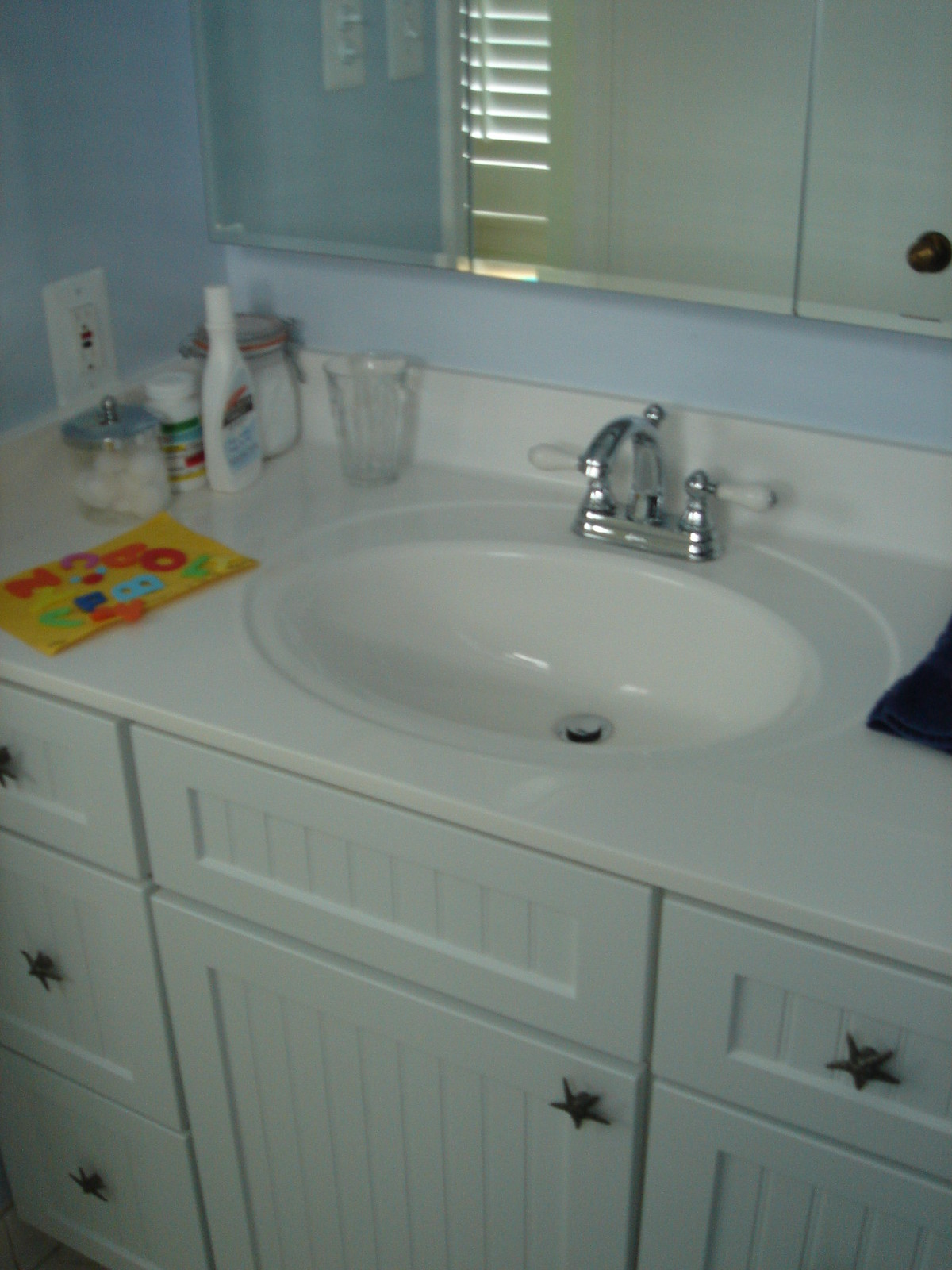A brightly lit bathroom features white cabinetry with distinctive vertical wood plank-style doors and bordered insets. The central section boasts two drawers above two doors, flanked by three additional drawers on the left. Each drawer is accented with bronze starfish-shaped knobs, adding a touch of coastal charm. The white ceramic countertop flows seamlessly into an integrated sink basin, complemented by a sleek, silver-colored faucet. The faucet handles are silver posts with white ceramic ends for a touch of elegance. A navy blue towel, partially cropped out of the image, is positioned to the right.

On the left side of the countertop, there is a yellow sheet of paper adorned with multicolored letters resembling refrigerator magnets in shades of yellow, blue, green, orange, red, and purple. Towards the back of the countertop, an assortment of items is neatly arranged: a bottle of cocoa butter lotion, an empty glass, a supplement-style pill bottle, and a glass canister filled with cotton balls topped with a metal lid. The bathroom's sky blue walls provide a refreshing backdrop, while a three-sectioned mirror above the sink enhances the room’s depth and brightness.